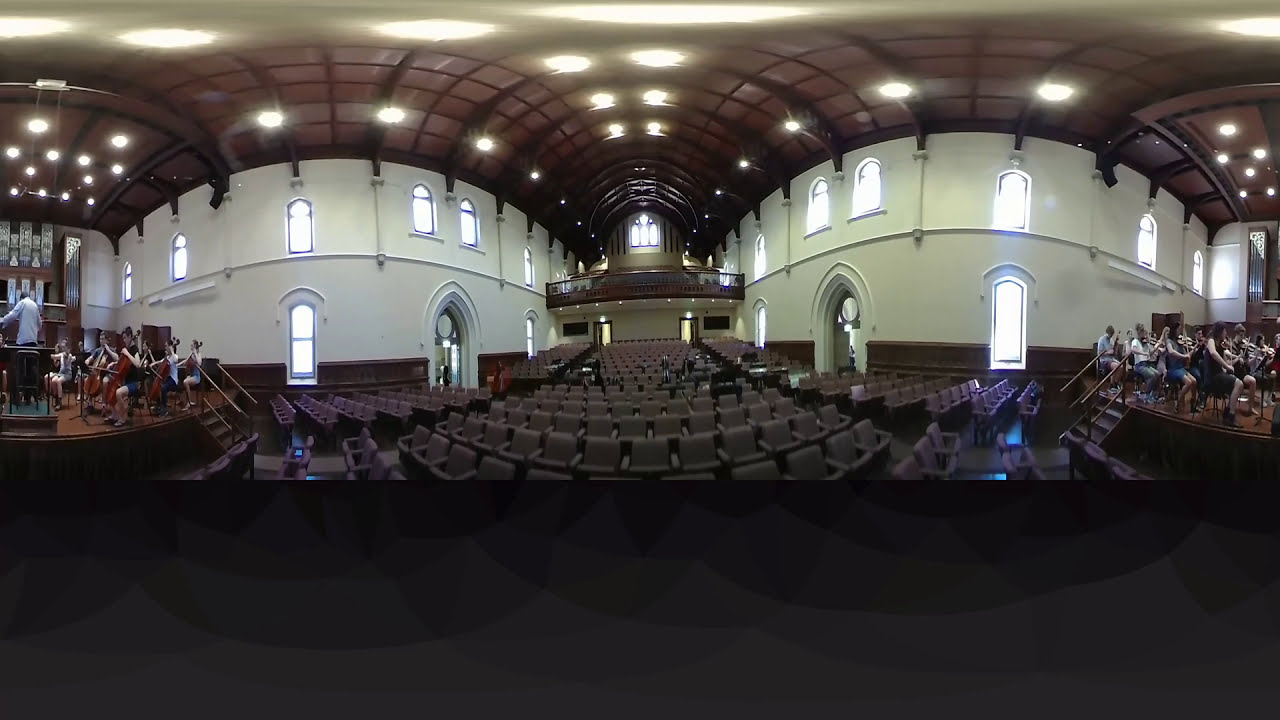The image depicts a vast auditorium, characterized by rows of predominantly empty, brown, cloth-covered fold-out chairs arranged in the middle and on the sides. The room is well-lit with circular lights affixed to both the ceiling and the walls, creating a soft white glow throughout the space. The auditorium's walls have a slight curve, adding to its expansive feel. 

At the front of the room, a stage hosts several musicians engaged in a practice session. On the right side of the stage, musicians are seated and playing violins and possibly other string instruments, while on the left side, another group plays larger string instruments like cellos or violas. A conductor stands on a small platform on the left, guiding the musicians with precise movements. The image appears to have been captured in a panoramic view, emphasizing the breadth of the auditorium and giving a slightly curved effect at the top and bottom. The overall scene conveys the meticulous details of a grand rehearsal in an expansive concert hall.